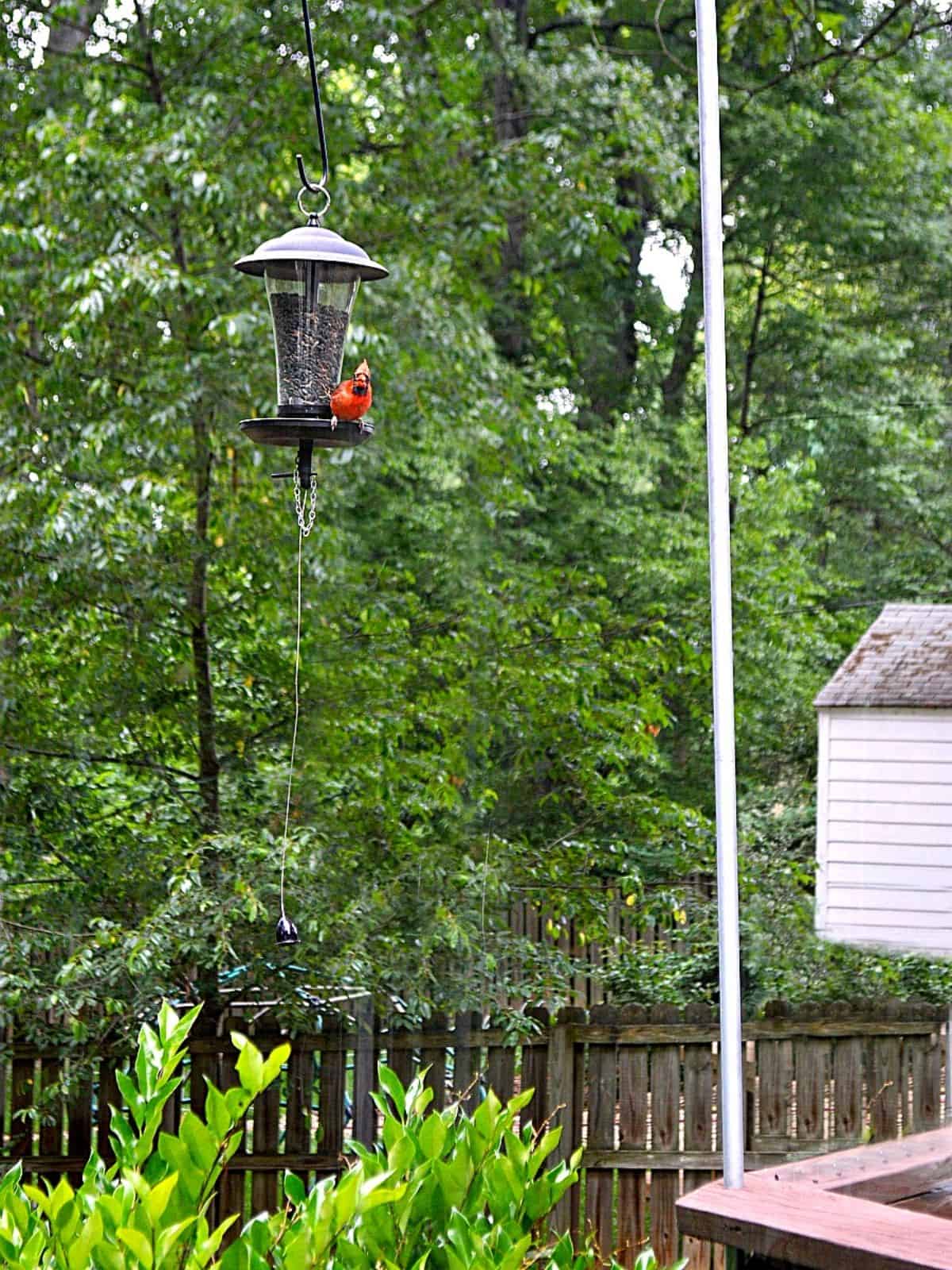In this detailed outdoor photograph, a black bird feeder is prominently featured. The feeder has a narrow top that widens into a cone shape and is topped with a lid. It hangs from a black shepherd’s hook and is situated near a white or silver pole on the right. A striking red cardinal is perched on the right edge of the feeder, its black facial markings around the neck and eyes clearly visible. Below the feeder, a white string dangles down to a black, bell-shaped object, and a small chain is attached to one of the feeder's lower perches. The feeder appears to be filled with black seeds, encapsulated within a glass cylinder that has saucer-like tops and bottoms.

Surrounding the bird feeder is a lush backyard setting. At the bottom of the image, vivid green plants contrast with a wooden fence. In the lower right corner, part of a wooden structure—possibly a porch or veranda—along with a long metallic pole is visible, extending beyond the frame. The background showcases towering trees with a mix of red, green, gray, brown, and dark green hues, and a glimpse of a house or garage peeks from the right side. The entire scene is captured during the daytime, presenting a vibrant and lively backyard atmosphere.